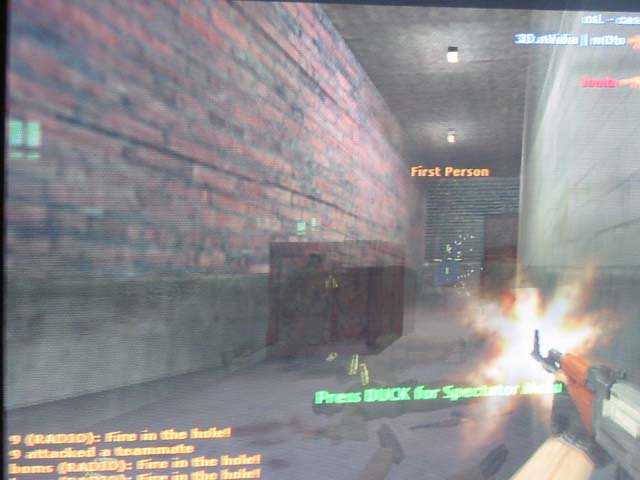A blurry screenshot captures a moment from a video game in first-person perspective. In the lower right corner, the player’s firearm, held by a hand near the tip, is visible. Green text near the top of the screen reads, "PRESS DUCK for spectator," though the exact wording is somewhat unclear due to the blurriness. Additional orange text is located in the bottom left corner. The background features a mix of red and gray bricks, indicating an indoor setting. A brown door and a section of black brick are at the top center. A large wooden crate is positioned slightly left of the center, dominating the foreground. No other characters are seen in this part of the game.